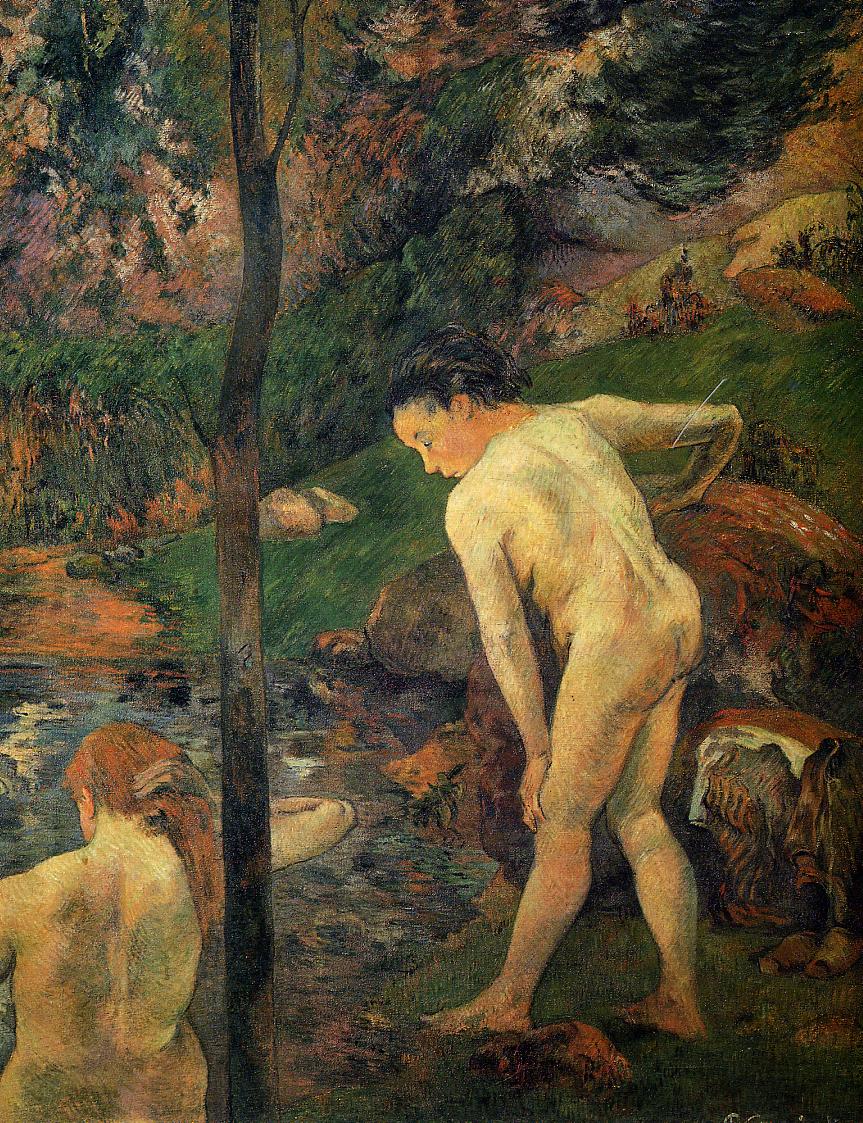This painting depicts a serene outdoor scene by a lake or pond, rendered in a vivid yet dark color palette brimming with hues of blue, green, purple, and brown. In the center of the composition stands a slender tree with a dark brown trunk and green, slightly purple-tinged leaves, towering upwards and dividing the painting. To the right of the tree, a naked man with dark hair bends over, one hand resting on his knee and the other on a hefty rock, his gaze downcast towards the water. On the left side, a woman with long, loose brown hair sits with her back partially turned, looking down towards the water. Both figures are unclothed, suggesting a moment of natural intimacy or bathing. The background features rock outcroppings and hilly terrain, reinforcing the natural setting. The water, with its reflective quality, mirrors the surrounding landscape, adding a tranquil element to the scene. The lower left corner of the painting subtly hints at faint writing, though it's obscured by darkness.